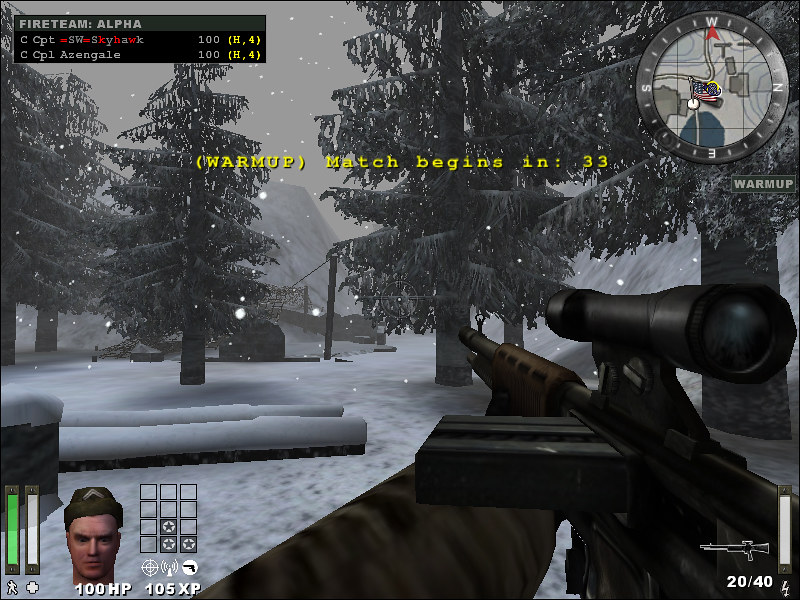A screenshot from a first-person shooter video game captures an intense moment where the player's character, dressed in long-sleeve camouflage attire, aims a sleek black firearm. The upper left-hand corner of the screen prominently displays the text "Fireteam Alpha," suggesting a mission or squad designation. In the bottom right-hand corner, the numbers "20-40" are visible next to a small image of a gun, likely indicating ammunition or a special weapon loadout. A navigational compass is situated in the upper right-hand corner of the screen, aiding in player orientation. Additionally, the lower left-hand corner showcases a small portrait of the player’s character, with a health indicator reading "100 HP" directly beneath it. The backdrop of this high-stakes moment is a serene yet treacherous snow-covered landscape, complete with towering mountains and dense clusters of evergreen trees, contrasting the tension of the virtual battlefield with the calm beauty of nature.